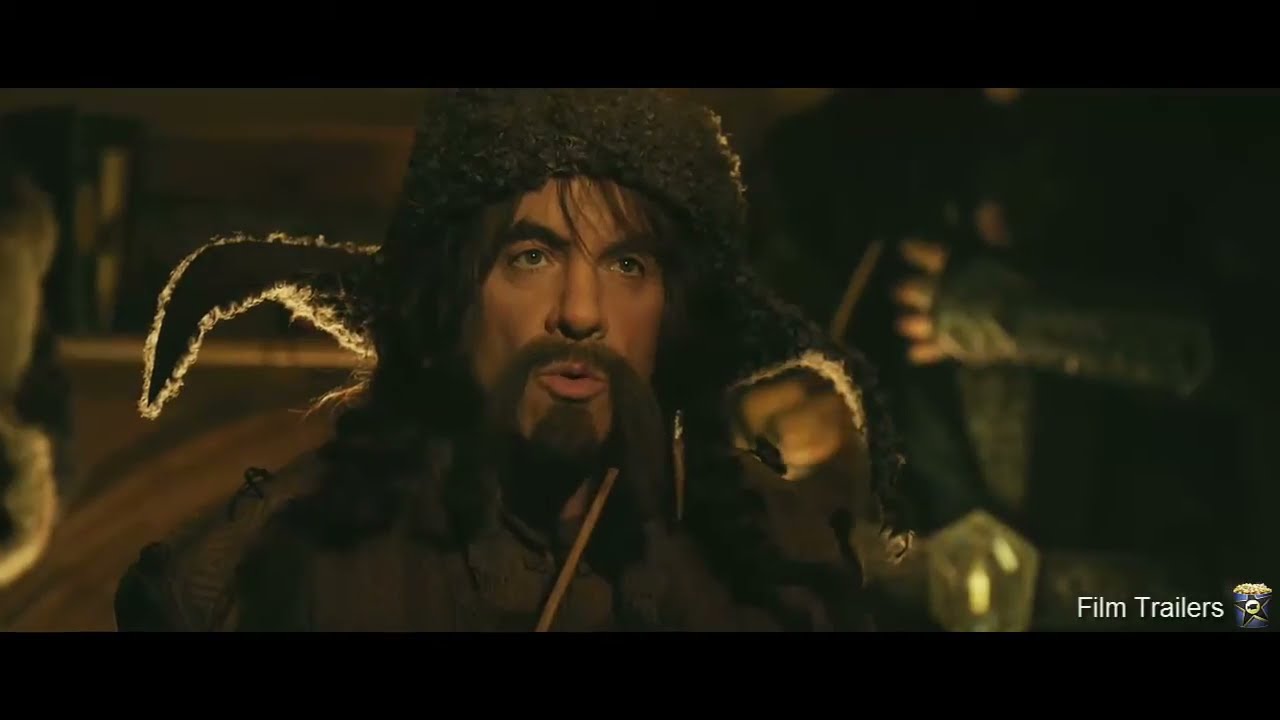The image is a still from a movie trailer, as confirmed by the text in the bottom right corner that reads "film trailers," accompanied by a small icon of a movie star over a popcorn bucket. The scene is set in a dimly-lit medieval or early modern setting, characterized by a predominantly dark and earthy color palette featuring shades of brown, gray, black, and subtle hints of white, yellow, and gold. 

At the center of the image is a handsome, warlike figure, depicted from the chest up. He has long, shaggy hair extending past his shoulders and is wearing a distinctive thick, dark woolen hat with ear flaps. The man's facial features include dark eyes, eyebrows, and a uniquely styled mustache that extends below his chin, along with a goatee. His lips are slightly parted as if he is in the middle of speaking, forming an "O" shape with his mouth. His attire is layered and dark, with a heavy jacket that signifies the historical period.

In the background, a second character is visible but obscured and blurry, with only part of his upper body and his hand on the central figure's chest discernible. The room's interior is dark, with an indistinct shelf carrying unidentifiable objects. A faint glow from a light source illuminates the scene from behind the primary figure, enhancing the dramatic and historical atmosphere of the setting.